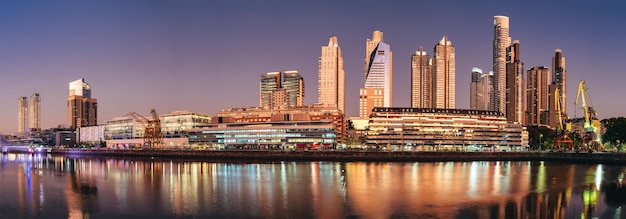This is a panoramic photograph capturing the twilight skyline of a large, vibrant metropolitan city. The sky above transitions from deep blue at the top to a gradient of dark purple, light purple, and finally light pink near the horizon. The cityscape is dominated by an array of illuminated high-rise buildings and skyscrapers, which are particularly dense from the right side to the middle of the image. Many of these buildings have balconies and numerous windows, reflecting their waterfront location. On the left side, there are a few distinct structures: two high-rise apartment buildings standing side-by-side, a tall brown building, and several shorter rectangular buildings. The right side features nine or ten more diverse high-rises with different materials, colors, and shapes, including some with pointed tops; a construction crane can also be seen amongst them. In front of this cityscape lies a calm body of water, which mirrors the city's bright, multicolored lights—yellows, reds, blues, and purples—creating a stunning, mirrored image on the water's surface. The city is separated from this tranquil water by what appears to be a seawall. The overall composition of the photo beautifully captures the serene yet vibrant essence of the city at twilight.